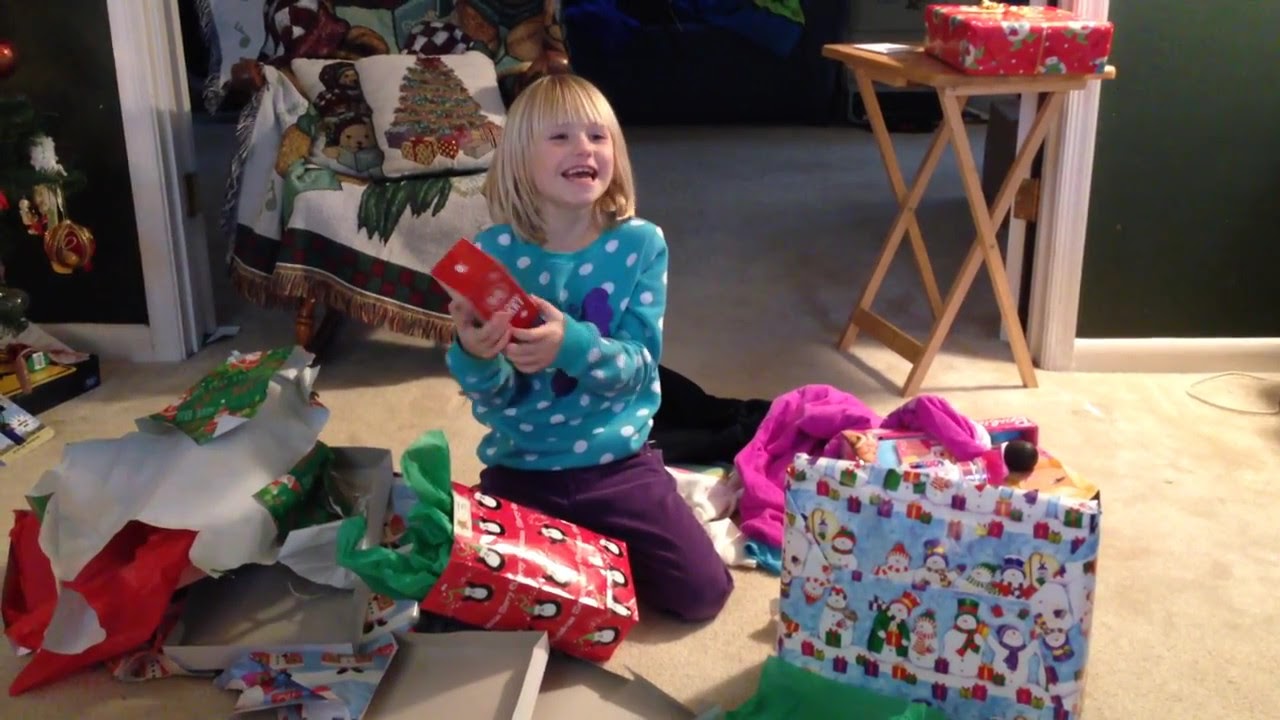In this warm, Christmas-themed living room, a very excited young blonde girl, approximately 7-8 years old, is joyfully opening her presents. She is kneeling on a cozy, fuzzy carpet, surrounded by a burst of red and green wrapping paper and various gift bags adorned with festive tissue paper. Clad in a blue shirt with white polka dots and purple pants, the girl gleefully holds up a red box that had been nestled inside a red bag filled with green paper. Behind her, a rocking chair draped with a blanket and several Christmas-themed pillows with tree and light bulb designs adds to the festive ambiance. In the background, a meal tray with another red present shares the space with a blue-wrapped gift and some already opened presents, including a pink article of clothing that might be pajamas. The scene is further enriched by the soft glow of warm lighting and the faint edge of a Christmas tree peeking into the frame, perfectly encapsulating the joyous spirit of the holiday.